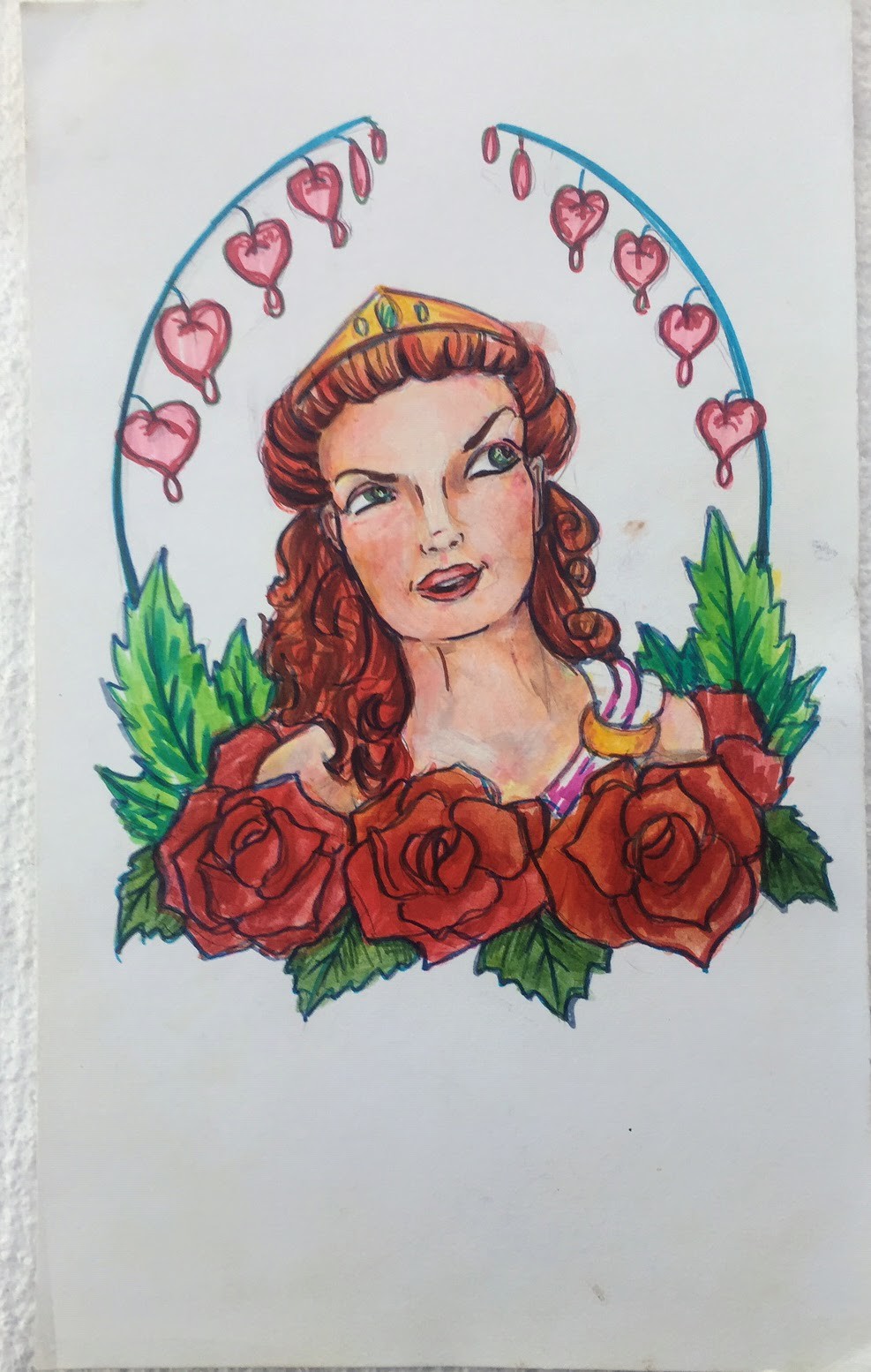This hand-created image depicts a striking woman with curly red hair, adorned with a regal gold crown set with green gems. Her dark brown eyebrows add to her expressive face, one arched with a slightly sinister air. She has piercing green eyes and faintly red lips. She wears a partially visible white collar with pink accents, complemented by a gold band near her shoulder. Above her head, there's a blue arch embellished with hanging red hearts, adding a whimsical touch. Her chest area is decorated with lush green leaves and vivid red flowers, with additional green foliage beneath them. Intricate details, such as the subtle wrinkles on her neck, enhance the realism of the artwork.